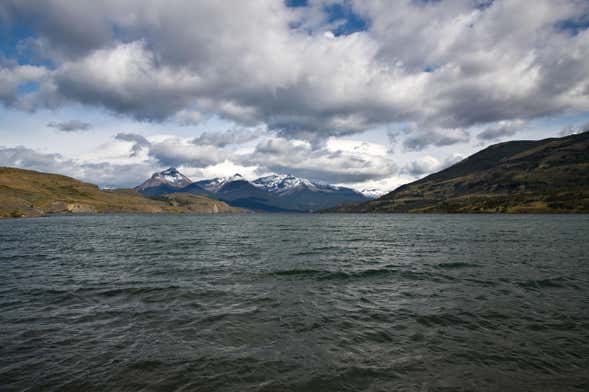The image depicts a dark naturescape dominated by a large, dark gray body of water that could either be a lake or an ocean, devoid of whitecaps but filled with dark, dank ripples. The bottom half of the frame is entirely water, creating a somber and somewhat desolate atmosphere. In the background on the right, there are ominous black hills, while the left side features greenish-brown hills. Far in the distance, snow-covered hills can be seen, adding a touch of brightness to the otherwise muted palette. Above this landscape, the sky is dark and overcast, with clouds transitioning to lighter hues and eventually a light blue sky in the far distance. The overall scene is strikingly bleak, with the dark water and hills contrasting sharply against the lighter sky.